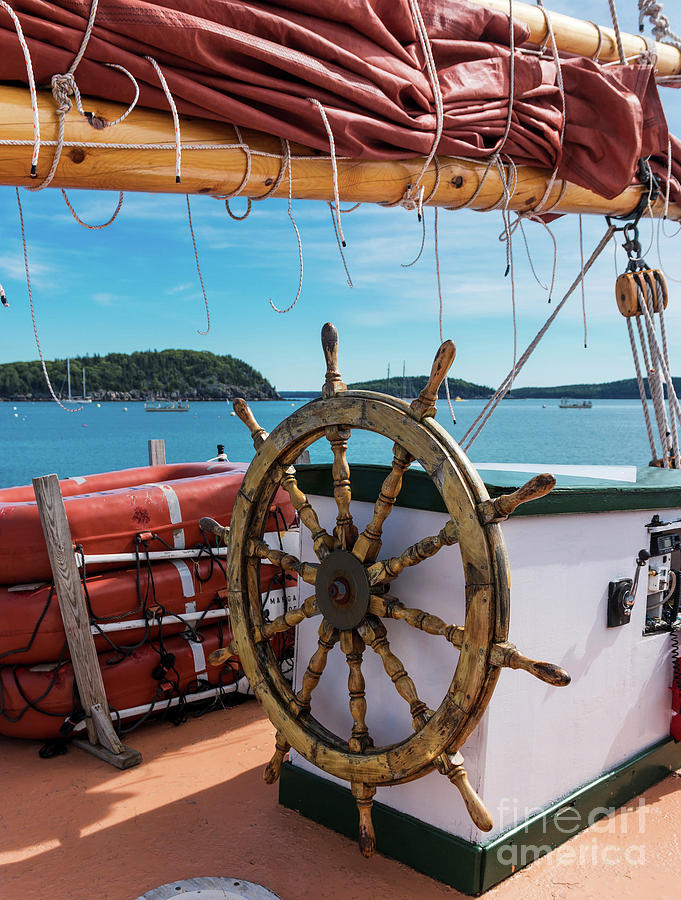This photo, taken from the cockpit of a boat, captures the scene from just behind the wooden steering wheel. The wheel, with its classic circular design and protruding spokes, is mounted on a platform that has a white central area flanked by green (or possibly black) borders. Adjacent to this is a wooden post supporting three orange lifeboats, a crucial safety feature. The background unveils a serene expanse of water with several small islands dotting the horizon. The sky above is a clear blue, lightly peppered with sparse, wispy clouds. Dominating the upper part of the image is the boat's sail, neatly rolled up between two long wooden masts. This sail is secured with ropes, ready to be unfurled when needed. Additionally, other boats can be spotted in the distance, adding to the nautical ambiance of the scene.